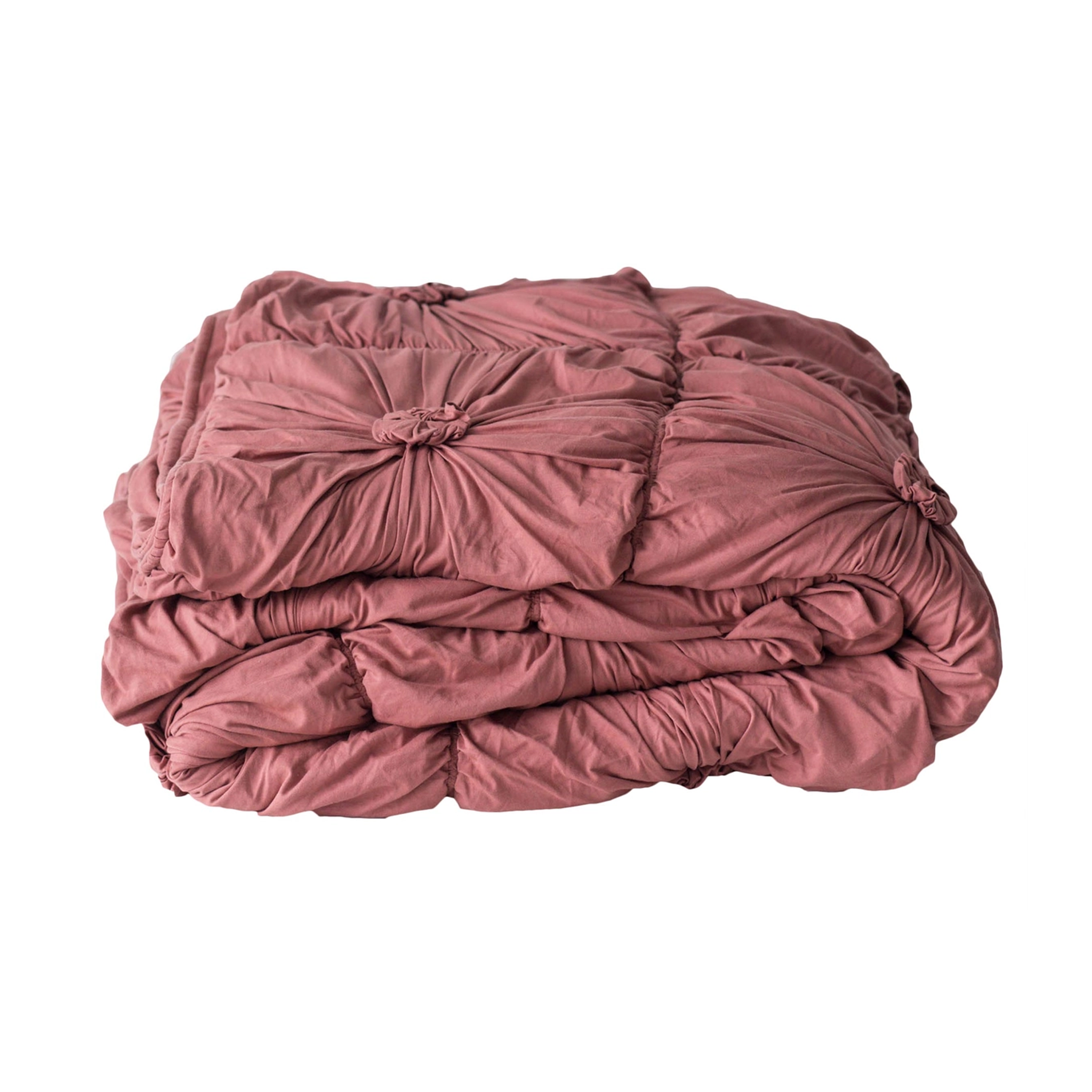In this detailed and centered image, a folded pink quilt-like blanket is the sole focus against a stark, solid white background. The blanket, positioned horizontally in the middle of the frame, appears to be folded multiple times, emphasizing its plush and voluminous texture. Its design features a series of pillow-like squares, each adorned with a small, gathered spot at its center, suggesting a handcrafted quality reminiscent of traditional quilts. The fabric exhibits numerous wrinkles and folds, lending a slightly unorganized yet cozy appearance. This image, devoid of any text, carries the essence of a stock photo showcasing a possibly homemade and cherished piece of bedding.